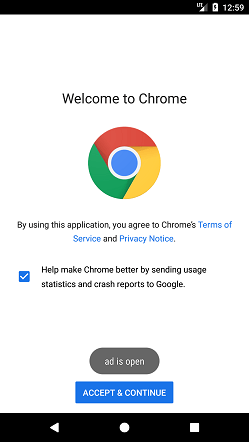The image captures a screenshot from a smartphone displaying the setup screen of the Google Chrome browser. At the very top, the phone's status bar shows the network signal, battery level, and time. Below the status bar, a white background prominently displays the message "Welcome to Chrome" alongside the Google Chrome logo. The text continues to inform users that "By using this application, you agree to Chrome's Terms of Service and Privacy Notice."

Further down, the screen asks for user consent to "Help make Chrome better by sending usage statistics and crash reports to Google," indicated by a blue checkbox that has already been selected. Following this, a gray box contains the option "Add is open." At the bottom of the screen, a blue button with the text "Accept and Continue" offers the user a way to proceed. The repetition of the "Welcome to Chrome" message and the associated terms underscore the importance of informed consent before using the application.